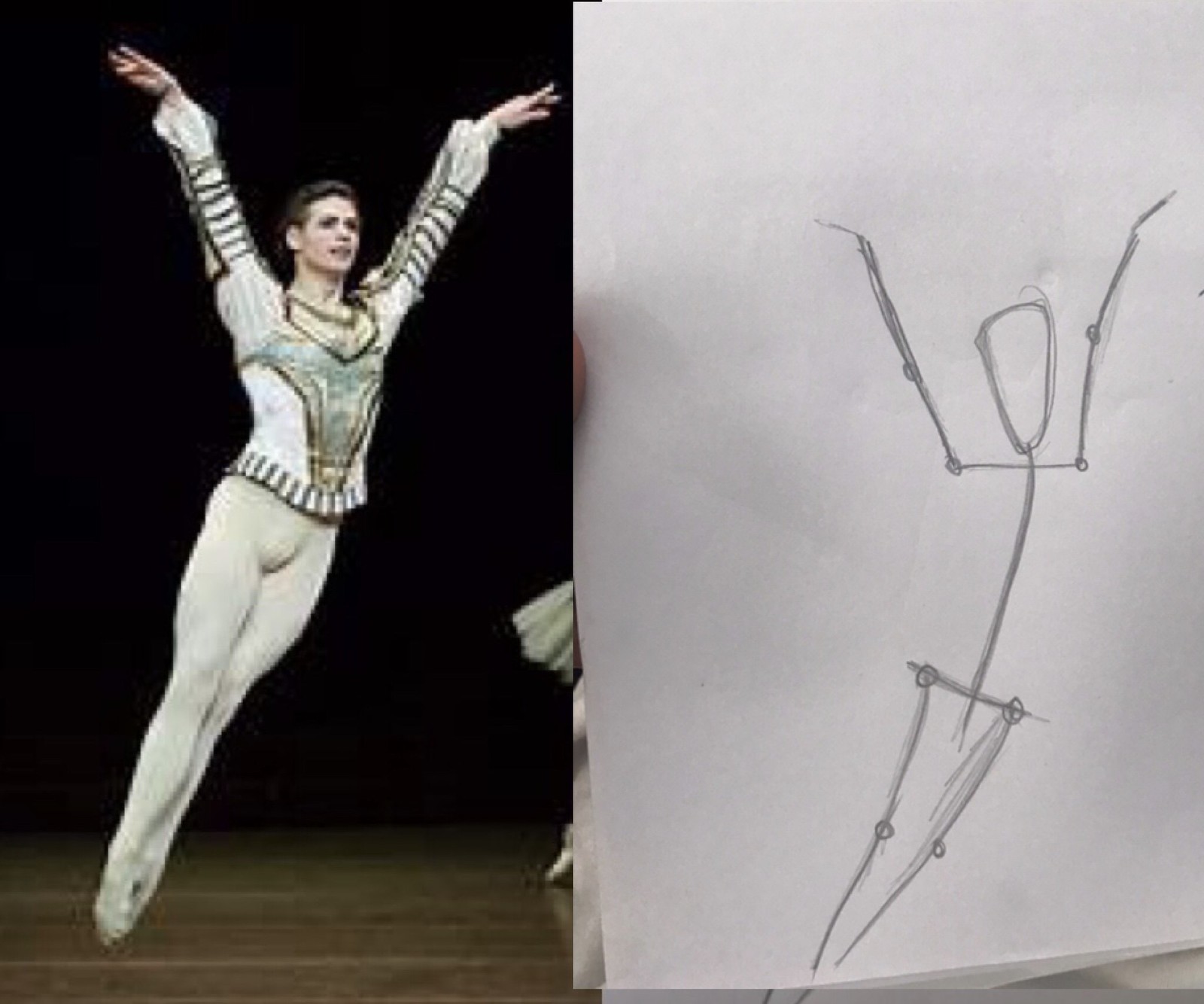In this image, two side-by-side visuals capture a dynamic ballet pose. On the left, a male ballet dancer is depicted mid-jump against a black background and a wooden floor. He has short dark hair and Caucasian skin. His arms are raised high above his head with his fingers elegantly spread, and his legs are together with toes pointed downward. He is dressed in white tights, and a long-sleeve white shirt adorned with a black V-shaped design across the chest, striped borders around the collar and sleeves, and additional striped patterns. To the lower right, part of a ballerina's white tutu and ballet shoe are visible, indicating her presence just outside the frame. On the right side of the image, a pencil drawing replicates the male dancer's exact pose with a simple stick figure. The stick figure has a circle for a head, straight lines for arms, shoulders, and legs, and a tiny part of a person's thumb is visible on the left edge of this white background drawing.